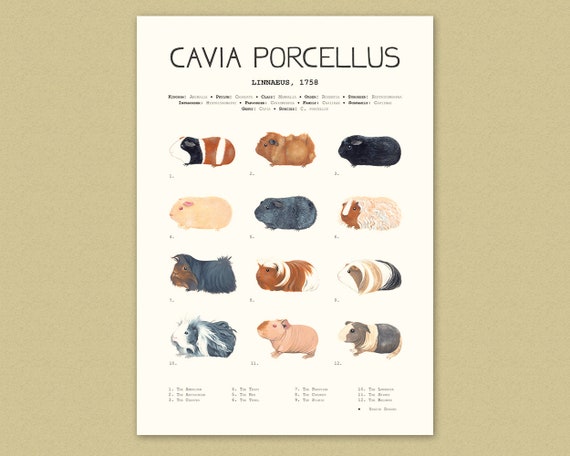The poster is an informative and visually detailed display titled "Cavia Porcellus," featuring an array of guinea pig illustrations. The poster, set against a light gray or tan background, has a white vertical rectangle layout. At the top of the poster, prominently printed in large black letters, is the species name "Cavia Porcellus," followed by "Linnaeus, 1758" in smaller text. Below the title, there are three brief lines of writing.

The main section of the poster showcases twelve detailed illustrations of different types of guinea pigs, arranged in four rows and three columns. Each guinea pig varies in color and pattern, demonstrating a rich diversity within the species. For example, the top-left guinea pig has a striped pattern with alternating hues of white, black, orange, and brown, while the subsequent guinea pigs exhibit colors such as full brown and full black. A couple of the animals appear to be adorned with accessories: the sixth guinea pig has a pink and white design, and the seventh features a blue covering that drapes over its head and sides.

Beneath each illustration, there are captions numbered from 1 to 12, likely identifying the differences or unique characteristics of each depicted guinea pig. Additional small text follows the last numbered caption, providing more context or information about the species. Overall, the poster combines scientific labeling with artistic representations to educate viewers about the variety within the species Cavia Porcellus.